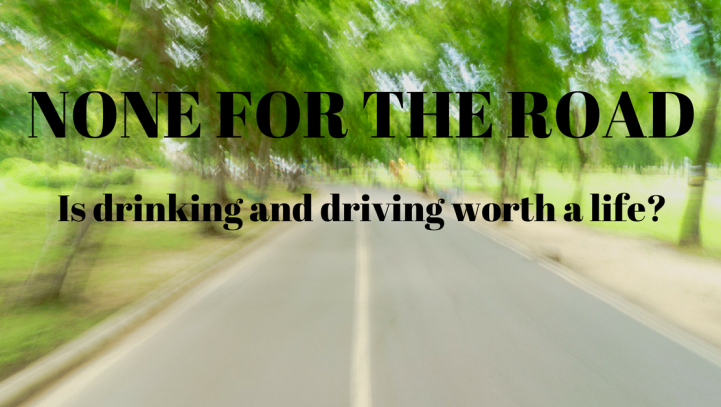The image appears to be an advertisement against drunk driving, featuring a highly blurred photograph that gives the impression of being taken from a moving car. The central focus of the image is a two-lane road with a yellow middle line, stretching straight into the horizon. Flanking the road are vibrant, lime-green trees and grass, creating a pastoral and serene scene despite the overall blurriness. The text superimposed on the image reads, "NONE FOR THE ROAD" in all-capital, bold black letters, with the phrase, "Is drinking and driving worth a life?" directly beneath it in smaller but equally bold black font. The blur effect suggests motion, reinforcing the dangers and consequences of drinking and driving. The entire scene exudes a sunny day ambiance, heightening the stark contrast between the idyllic setting and the grave message conveyed by the ad.